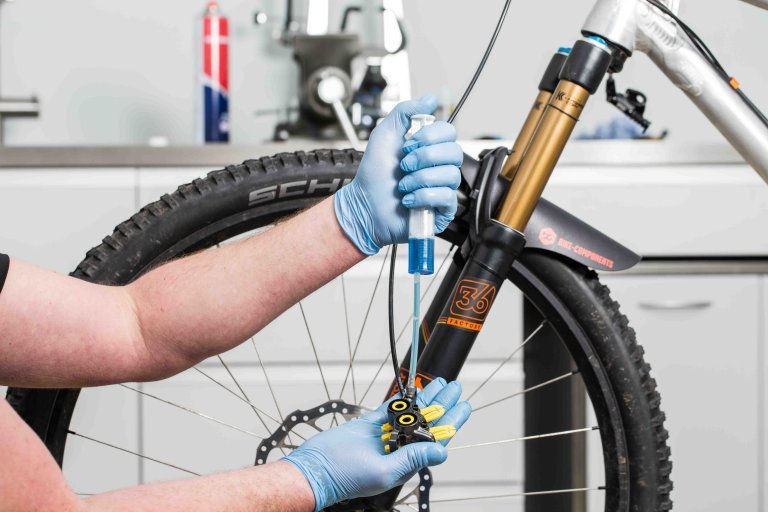In a brightly lit indoor workspace with white cabinets and a cluttered workbench, a European, likely Caucasian individual can be seen meticulously performing a maintenance task on a bicycle. Wearing blue latex gloves, they are using a plastic syringe-like device to inject a blue liquid, possibly brake fluid, into a mechanical component of the bike. The bike, notable for its golden and silver accents, features a black and yellow part with orange text reading "36 Factory." The identifiable elements include the front wheel and a distinct gold-colored metal piece leaning over it. Bare arms hint that the person might be wearing a short-sleeved shirt. Surrounding the scene are various tools and items on the countertop, including a red and blue aerosol can, highlighting the environment's functional and practical nature.